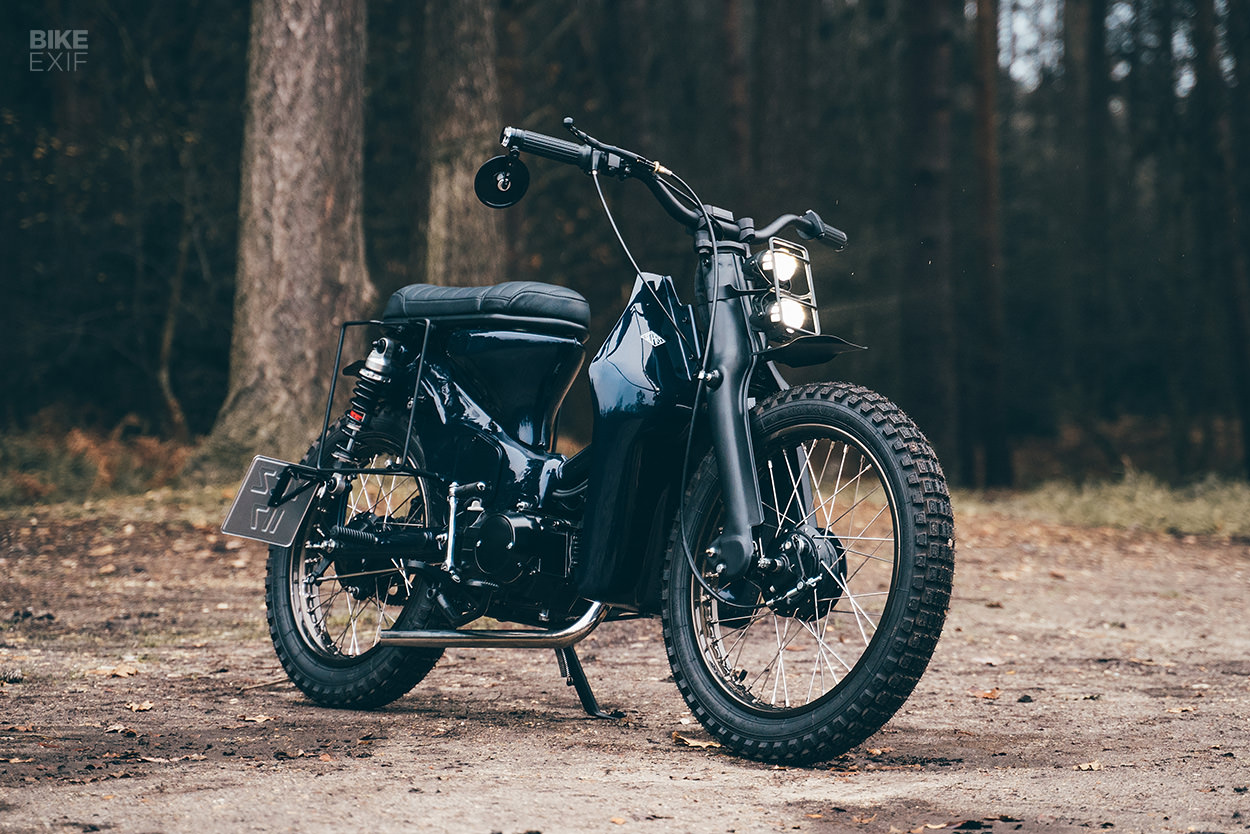The image captures a sleek, all-black motorcycle with silver accents set in a wooded, forest-like area. The horizontal photo, taken outdoors on a patch of dirt and some grass, shows the motorcycle angled to the right. Prominent features include two headlights stacked vertically just below the handlebars, a mirror hanging from one handlebar, and a visible license plate reading "bike exif." The motorcycle rests on its kickstand with shiny black bodywork, black tires with silver spoked wheels, a black leather seat, and a chrome exhaust pipe. A large shock absorber descends from behind the seat. The background is densely wooded, with trees of varying shades of green, gray, and brown stretching across the entire width of the image and extending out of the frame at the top. There are no people present in the photograph.